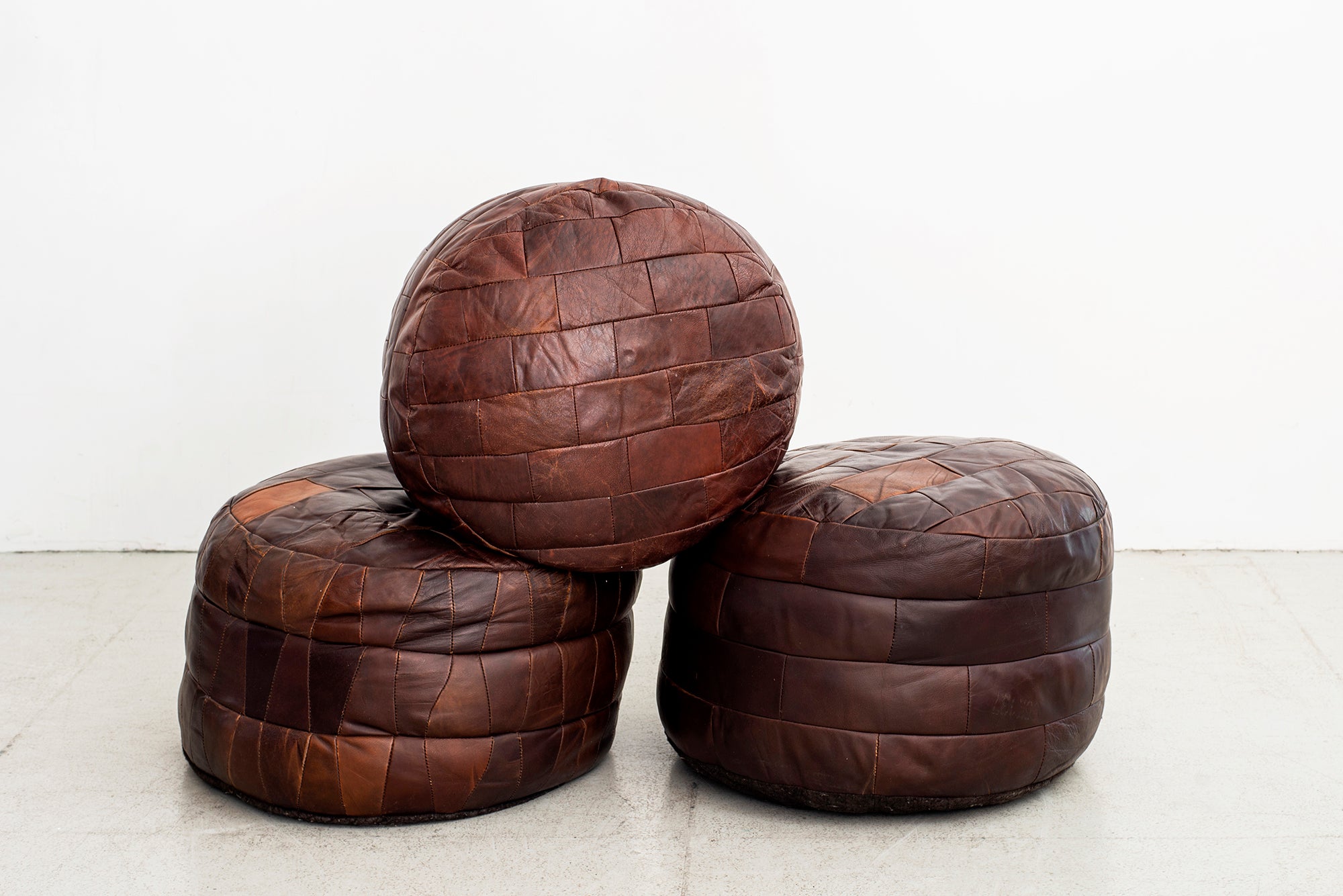In a minimalist setting, three leather poufs, resembling beanbags, are arranged against a plain white wall with off-white linoleum flooring showing some dirt at the baseboard. These poufs are made of patchwork leather pieces, giving them a textured, brick-like appearance, characterized by a worn medium sheen in various shades of brown, dark brown, grey, and hints of dark purple and orange. They form a small pyramid, with two poufs standing upright on the base and another one placed on its side atop them. Each pouf is circular and cylindrical, roughly the size of a footstool, no bigger than 24 by 24 by 24 inches, providing a compact yet distinct seating arrangement in the scene.